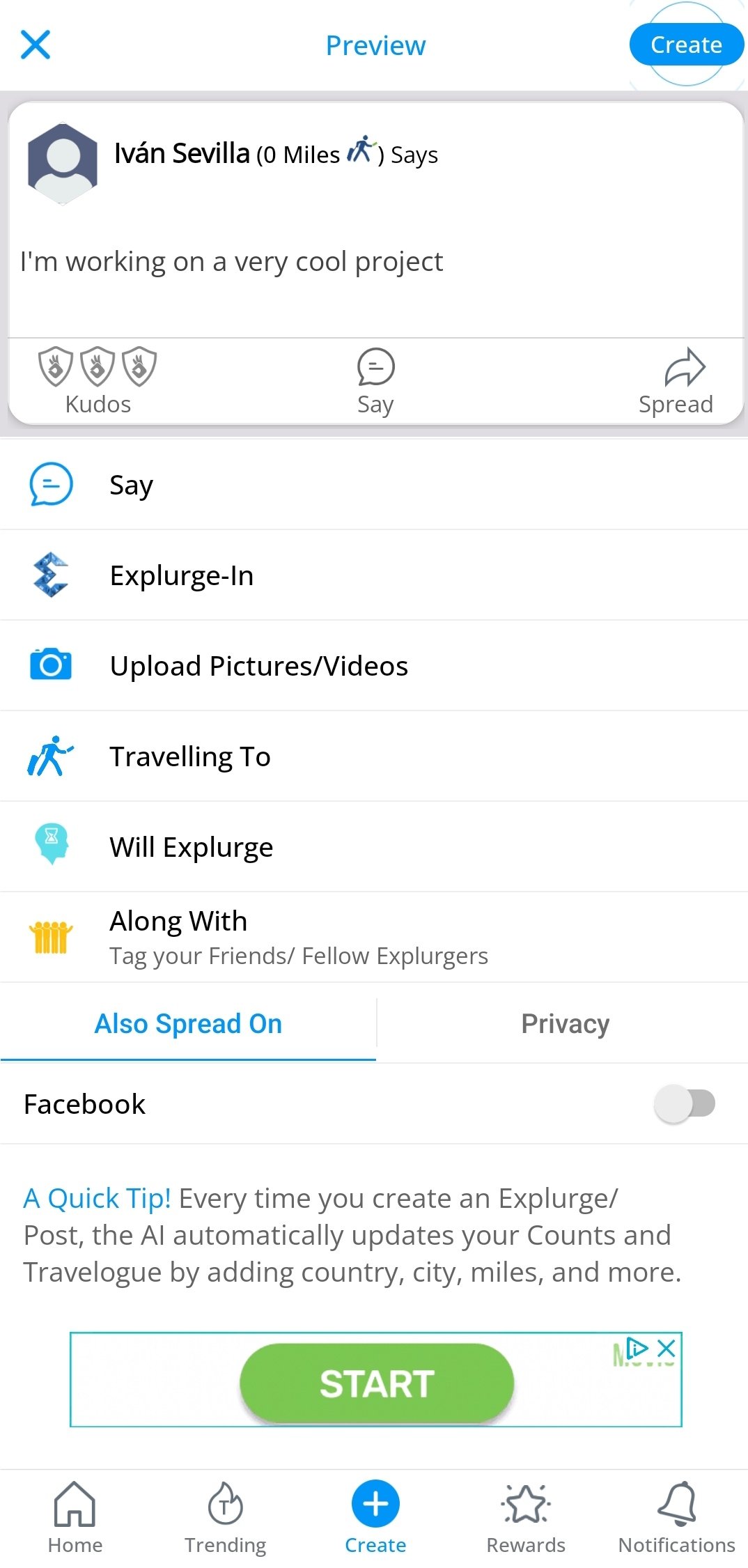This image is a screenshot from a cell phone, characterized by its narrow and tall display. The screen depicted is an unfamiliar interface for updating and inputting information into Facebook. At the top of the screen, there are three significant elements: an X button for closing, a preview hyperlink to preview the content, and a create button to initiate a post.

Below these buttons, within a gray rectangle, there is a message from a user named Ivan Sevilla, which reads: "I'm working on a very cool project." Adjacent to his message are options that allow you to reply, share the information by posting it, or give kudos to Ivan for a job well done. 

The interface provides a variety of options for updating your status. It lists actions such as "say something," "explore gin," "upload pictures," "travel to," and more, including tagging friends.

Toward the bottom, there is a Facebook disclaimer and a quick tip for users. The screen concludes with a prominent green "Start" button, featuring the word "Start" in bold white font.